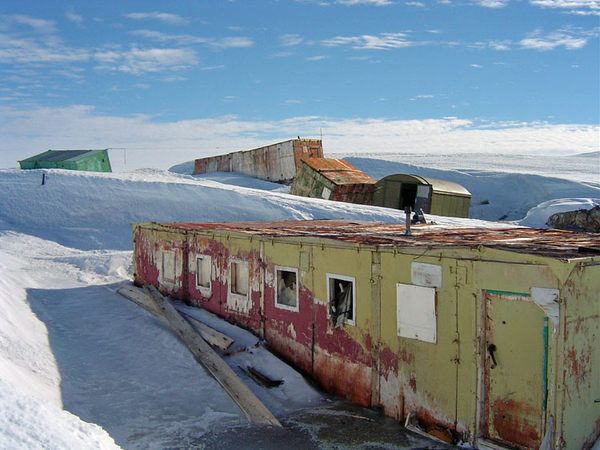The photograph captures a desolate, snow-covered outpost, possibly in the Arctic or Antarctica, showcasing a series of dilapidated structures scattered unevenly across the icy terrain. In the foreground stands a prominent container building with a red top and a façade bearing splotches of red, beige, and green paint. This worn-down structure is partially rusty and features a door and windows, surrounded by two large wooden planks on the ground to its left.

Towards the background, a green container building is visibly tilted, accompanied by another rusted, white structure that leans slightly upward. To the right, a smaller gray and red building sits, adjacent to a relatively newer, more intact shed with a teal and brown exterior, blending like the color of grass. Snow-covered hills flank the scene on both sides, and the horizon stretches into a cyan sky adorned with wispy white clouds, suggesting a time of morning or midday. The outpost's overall abandoned and rusting state, with open doors and sunken containers, hints at its former life as a research center now left to the mercy of the harsh, icy landscape.